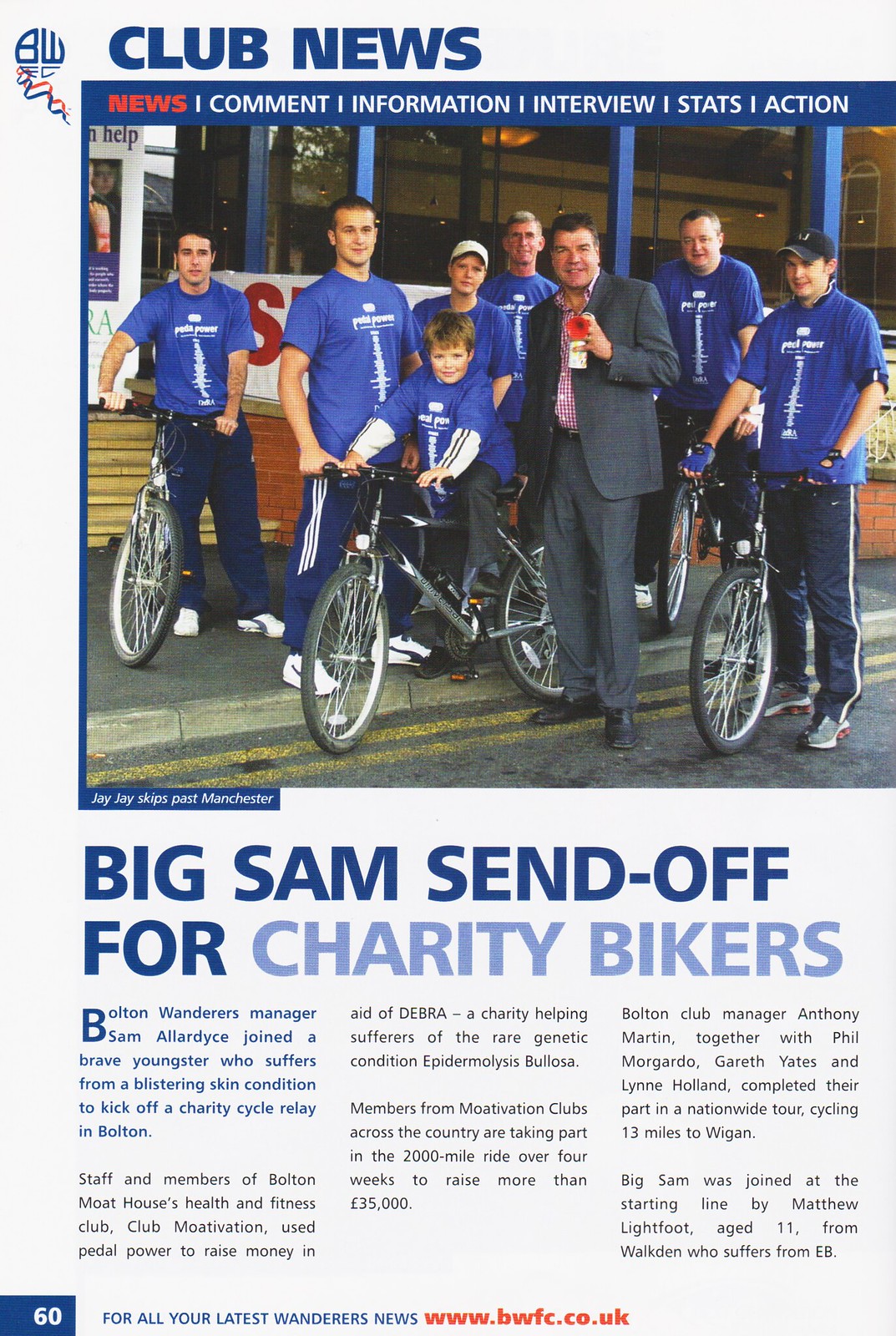This poster, titled "Club News," has a blue header and features prominent red words: News, Comment, Information, Interview, Stats, and Action. Below this header, there is a large image of a man in a gray suit, with a group of people wearing blue shirts and long pants riding bicycles next to him. The title of the main article, "Big Sam Send-off for Charity Bikers," is written in lighter blue. The article details Bolton Wanderers Manager Sam Allardyce, who joined 11-year-old Matthew Lightfoot, a brave youngster suffering from the rare genetic skin condition epidermolysis bullosa (EB), to kick off a charity cycle relay in Bolton.

The charity event was organized by Bolton Mote's House Health and Fitness Club, part of the Motivation Club network. They aimed to raise over £35,000 in aid of the charity DEBRA, which supports those afflicted by EB. Members from different Motivation Clubs across the UK participated in the extensive 2,000-mile relay, which lasted four weeks. Key participants included club manager Anthony Martin, Phil Margardo, Gareth Yates, and Lynn Holland, who each cycled 30 miles over a weekend. The poignant kickoff was symbolized by the presence of Big Sam and young Matthew, rallying support for a meaningful cause. At the poster’s very bottom, the number "60" is listed in the lower left corner, followed by a call to action: "For all your latest Wanderers news, visit www.bwfc.co.uk."